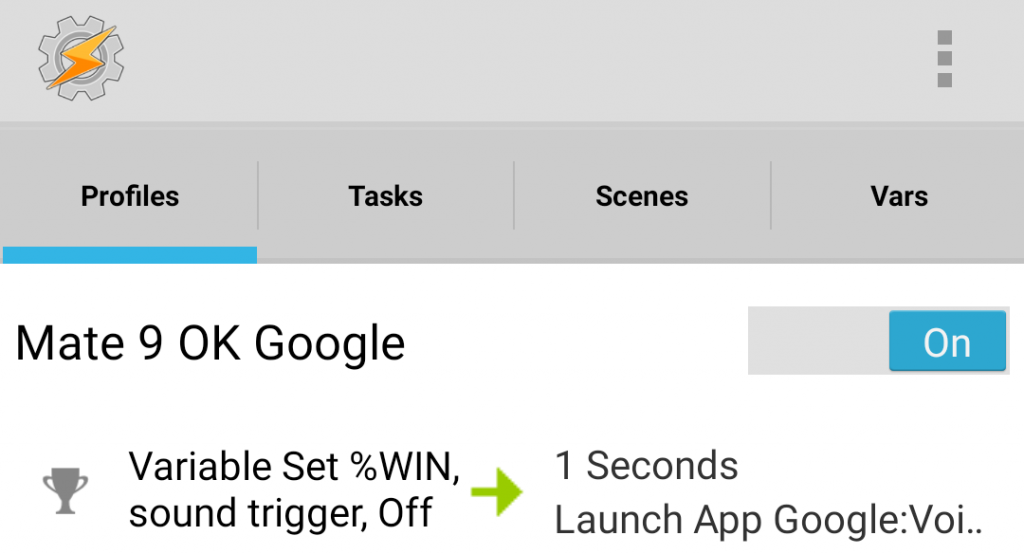This screenshot displays a detailed and organized interface segmented into several distinct sections. 

At the very top of the image is a long, narrow, two-tone gray rectangle. The upper part of this rectangle is light gray, and in the upper left-hand corner, there is an icon of a gear that contains an orange lightning bolt symbol, suggesting a settings or configuration option possibly related to power or charging. On the right-hand side of this top rectangle are three stacked, darker gray boxes.

Beneath this lighter gray rectangle is a slightly darker gray bar divided into four labeled sections: Profiles, Tasks, Scenes, and Vars. The section labeled "Profiles" is highlighted with a bold blue line underneath it, indicating it is the currently active or selected tab.

Transitioning down from the gray section, the background color changes to white. On the left side, in black text, it reads "Mate 9 OK Google," which appears to be an identifier or command prompt for a Google Assistant device or service. Within the same row but on the right side, there are two adjacent rectangles, with the sides touching in the middle. The left rectangle is light gray, and the right rectangle is blue, containing the white text "On."

Below this, on the left, there is a small icon of a trophy next to a line of text that reads "Variable Set Percent Win Sound Trigger Off." On the same line further to the right, a lime green arrow points to the right, leading to the text "One Seconds Launch App Google VOI," which seems to be a sequence command or task instruction, indicating a one-second delay before launching a Google Voice application.